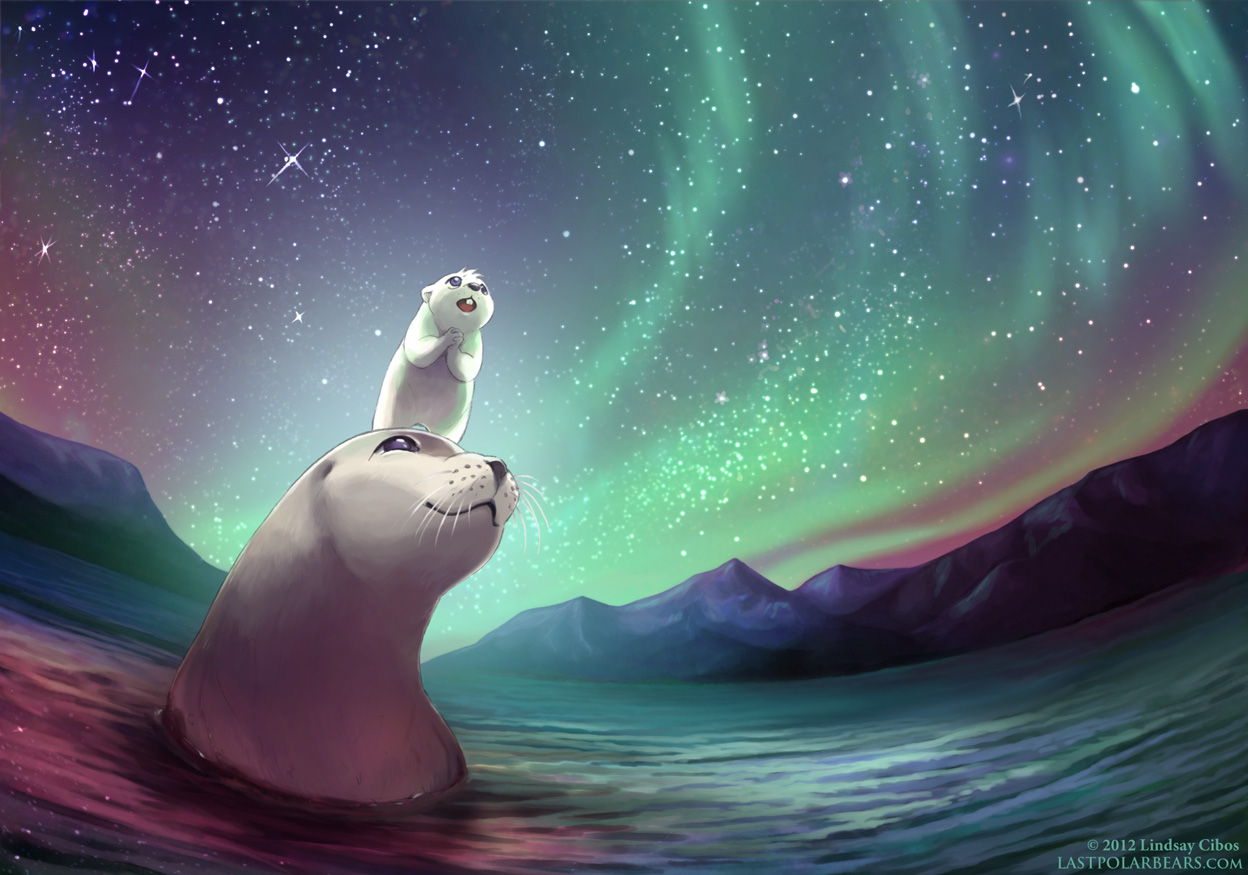This digital illustration by Lindsey Seboos, signed in teal text in the lower right corner with "2012 Lindsey Seboos, Lastpolarbears.com," captures a mesmerizing nocturnal scene in the wilderness. It features a happy, silver-gray seal with a white nose and black eyes, poking its head and neck out of a shimmering ocean that reflects the ethereal colors of the Northern Lights. On top of the seal's head stands a small, white-furred, gray-bellied mouse with buck teeth, its front flippers together and mouth open in apparent delight.

The background is dominated by a breathtaking display of the Aurora Borealis, with swirling green, purple, and teal lights illuminating a dark navy and purple sky sprinkled with twinkling stars. This celestial spectacle bathes the entire scene in a magical glow. The horizon is framed by mountains on both the left and right, adding depth to the composition. The ocean beneath the seal transitions from purplish hues on the left to greenish and teal on the right, further enhancing the enchanting atmosphere of this night under the Northern Lights. This meticulous and whimsical artwork evokes a sense of wonder and highlights the beauty of nature.